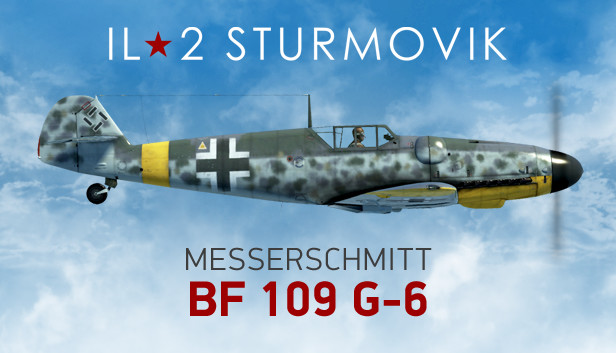The image is a detailed render, possibly derived from a video game, showcasing a World War One-style fighter plane flying in a blue sky dotted with clouds. The plane features a camouflage design with a mix of dark olive, lighter green, and gray-green tones interspersed with white. Its tip is marked in black, and the underside is yellow. Notable details include a black and white iron cross on the plane's left side, adjacent to a yellow stripe. The plane has a single black wheel visible beneath the tail fin. Above the aircraft, white text reads "IL," followed by a red star and "2 Sturmovik," while below, gray and red text spells out "Messerschmitt Bf 109 G6," indicating the model of the plane. Through a window, the silhouette of a single pilot can be seen inside the cockpit.